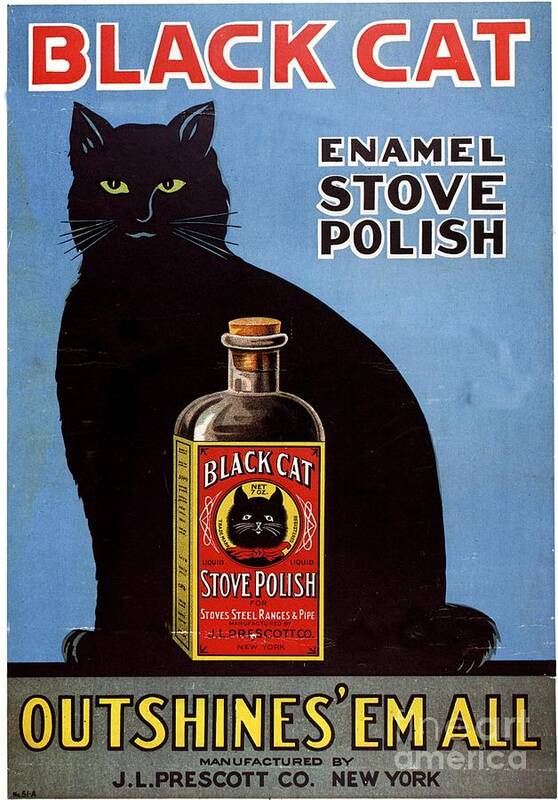The advertisement predominantly features a vibrant blue background at the top, accentuated by bold red and white outlined text that prominently reads "BLACK CAT" in all capital letters. On the right side of the advertisement, it mentions "enamel stove polish" in a mixture of black and white text. Centered in the image is a striking black cat with piercing yellow eyes and distinct black whiskers.

In front of the cat, there is a bottle of the product prominently displayed. The bottle is labeled "Black Cat" and specifies the net weight of 7 ounces (7 oz). The label also indicates the product's usage, listing "stove polish, stove steel ranges, and pipe." 

At the bottom of the advertisement, a grey banner features the text: "How shines them all," written in yellow. Additionally, the banner states, "Manufactured by J.L. Prescott Co. New York," confirming the manufacturer's details in black typography. The overall composition effectively combines specific product details with visually striking imagery to capture attention.